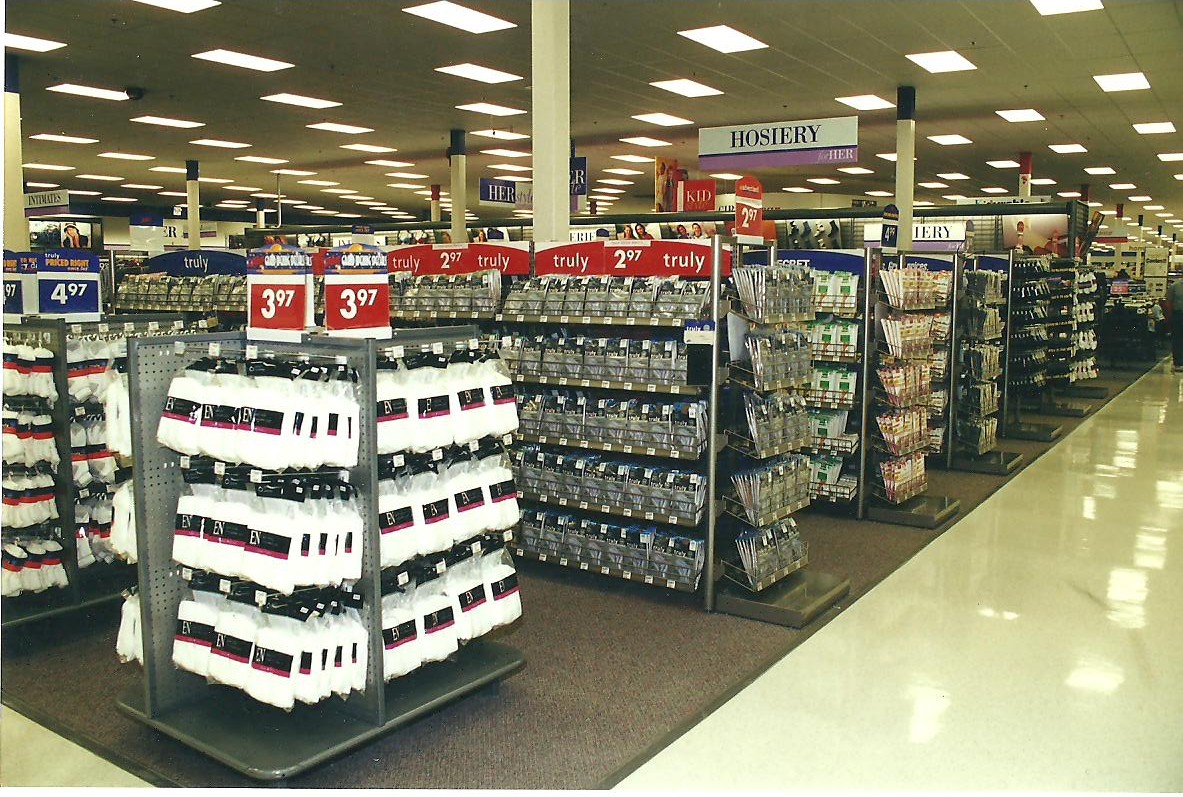This image depicts the interior of a brightly lit department store, specifically in the hosiery section. The store specializes in various types of clothing, predominantly featuring socks, underwear, and tights. There are multiple square stands displaying these items, and each stand is labeled with large, prominently displayed price tags. The prices are notably low, with red tags showing $3.97 and $2.97 and blue tags indicating $4.97. The merchandise primarily consists of repetitive displays of white and dark-colored items, with minimal variation. Fluorescent lights illuminate the space, their reflections visible on the linoleum floor, and there are no people present in the scene.